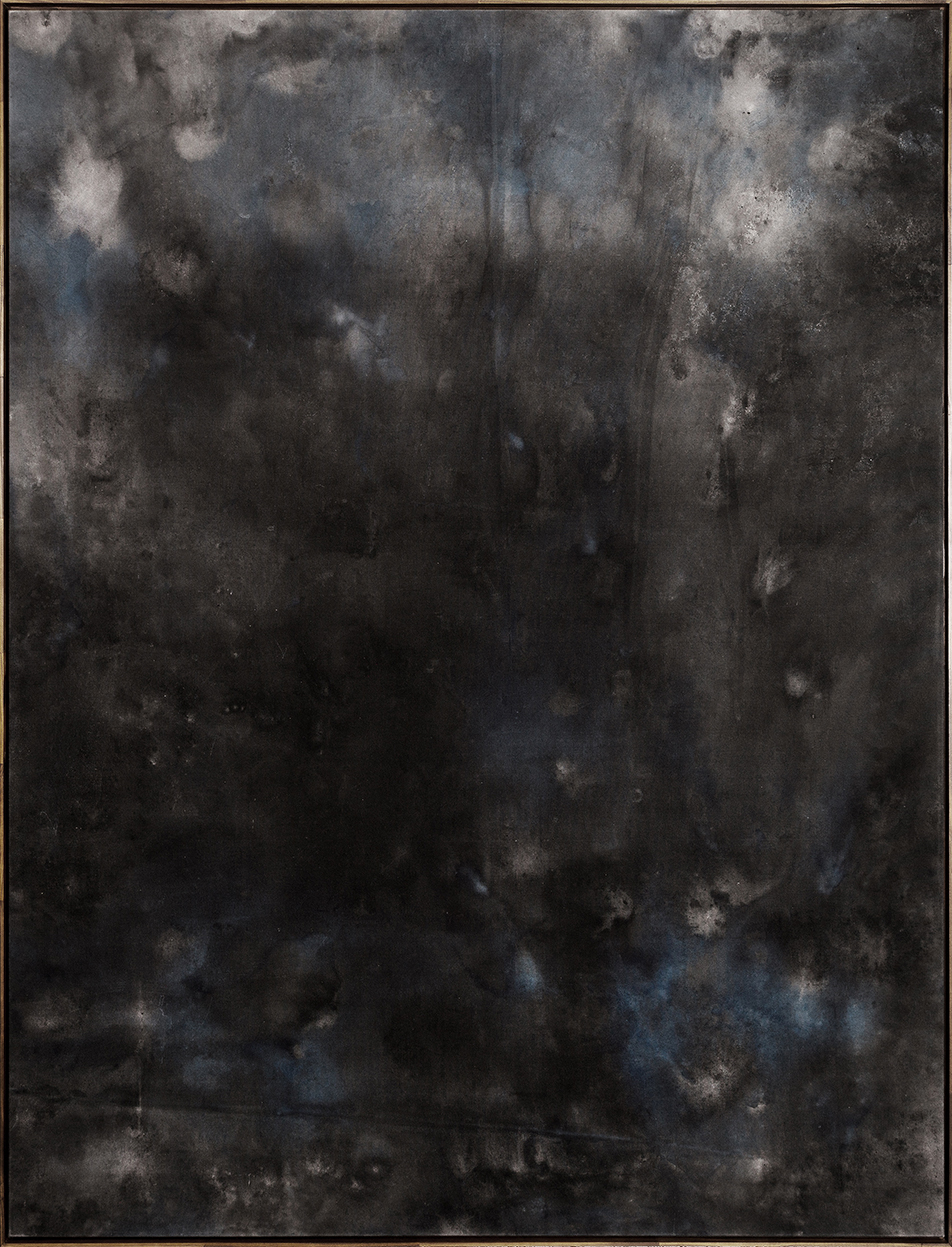The painting is an abstract composition dominated by dark, shadowy hues, primarily in black and grey tones, with accents of white and blue. The scene evokes a stormy night sky, characterized by brooding clouds interspersed with occasional light shining through. The top part of the painting appears brighter, with light grey and white hues suggesting patches of light peeking through dark clouds. In contrast, the lower portion features deeper black tones with some hints of blue.

Throughout the image, smudges and streaks create a sense of movement, as if meteors are falling from the sky or water is cascading. The middle part is punctuated by small, black bead-like spots, adding to the texture. The mingling colors form no distinct shapes, offering instead a sense of fluid, watery abstraction. The canvas is consistently dark, with lighter and darker areas that give depth and dynamism to the composition.